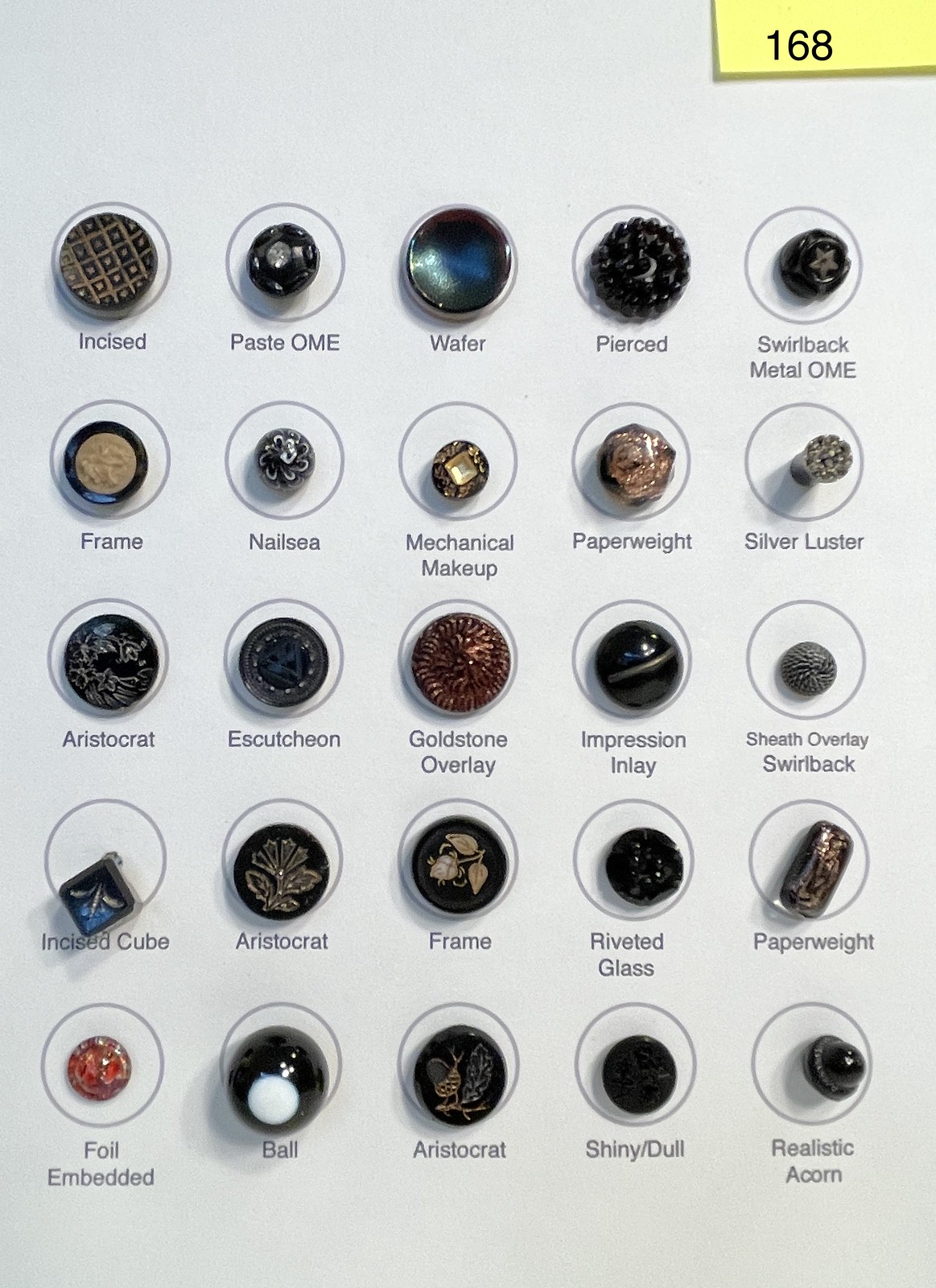This rectangular photograph features a detailed display of intricately designed stones arranged in a 5x5 grid against a light blue background. Each of the 25 stones is placed inside a black circle with its name inscribed below in black text. The stones vary in design and color, including black, bluish, and brownish hues, with some displaying a striking shine. The stones exhibit different textures and patterns, such as a black and gold checkered incised stone, a smooth blackish-blue wafer, and a black textured pierced stone.

Prominent names among the stones include:
- Incised 
- Paste-on 
- Wafer 
- Pierced 
- Swirled back metal-on 
- Frame nail-C 
- Mechanical makeup 
- Paperweight 
- Silver luster 
- Aristocrat 
- Astute geon 
- Goldstone overlay 
- Impression inlay 
- Shield overlay 
- Swirled back 
- Incised cube aristocrat 
- Frame 
- Riveted glass 
- Foil embedded 
- Bowl 
- Aristocrat shiny 
- Dull 
- Realistic 

In the upper right corner of the image, there is a small yellow strip with the number "168" printed in black, which resembles the edge of a piece of paper. This image presents a meticulous arrangement of various designer stones, each uniquely crafted and labeled for identification.